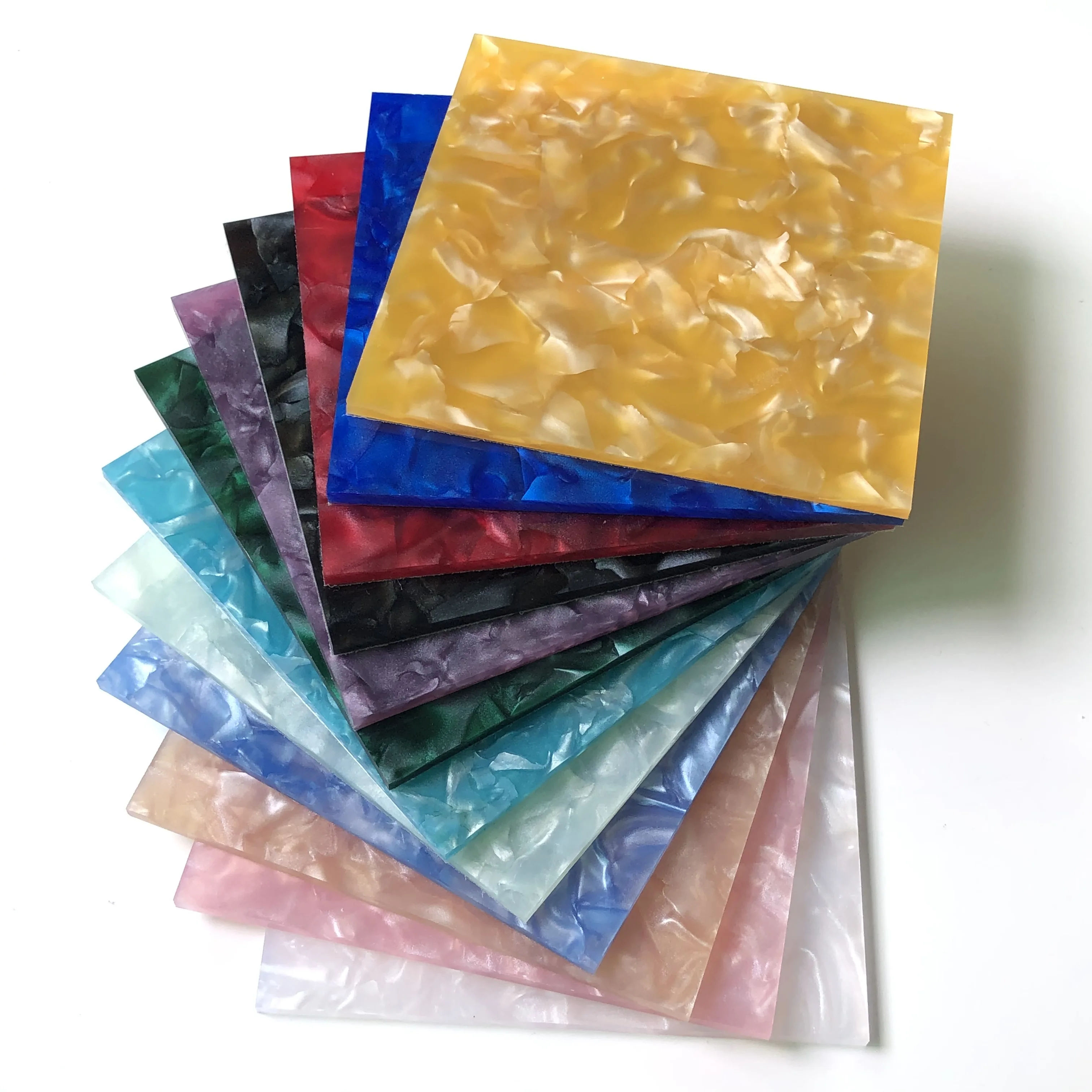This image showcases a set of twelve square tiles arranged in a fanned-out stack on a pristine white background, likely in a studio setting with a light source casting a shadow to the right. Each tile, featuring distinct marble-like wavy textures and a smooth finish, displays a unique color palette. From top to bottom, the colors of the tiles include vibrant gold, deep navy blue, rich dark red, classic black, elegant purple, refreshing dark green, soft light teal, pale light blue, a silvery pearlescent hue, striking dark purple-blue, inviting peach, delicate pink, and pristine white at the bottom. The intricate marbling and color variations add depth and interest to each tile, creating a captivating visual composition.